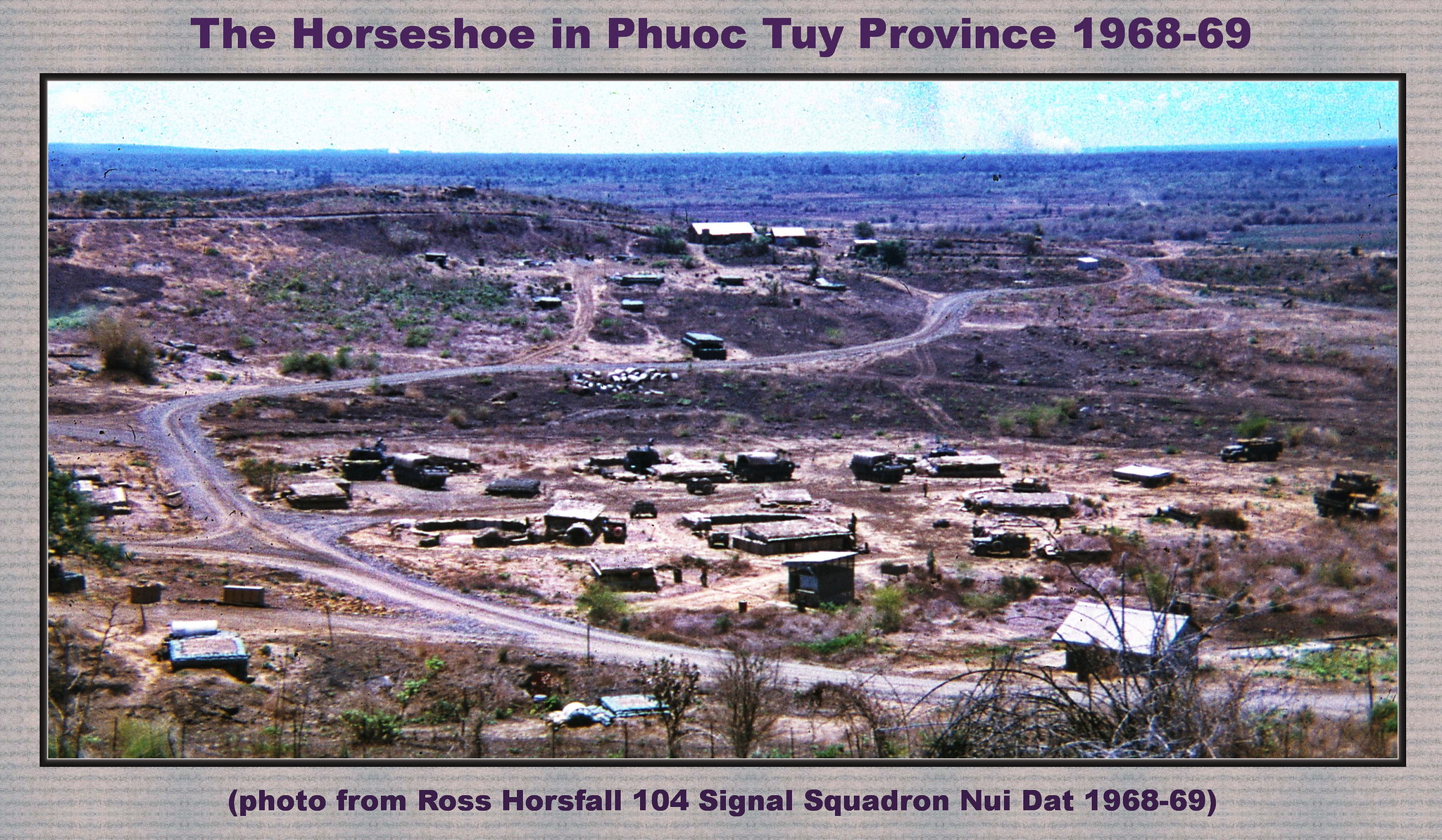This is a color photograph dating back to the Vietnam era, specifically between 1968-1969, featuring the arid, desert-like landscape of Fort Hoi Province. The image showcases a barren, rural area with sparse vegetation, consisting mainly of weeds and bushes scattered throughout. There is an unpaved road cutting through the scene, with a few huts, vehicles, and pieces of equipment dotting the foreground. The horizon stretches far into the distance, meeting a flat expanse of fields under a hazy, dark gray, and somewhat white sky. The photograph is bordered by a tan outer frame and a black inner frame. The top of the tan border is inscribed in purple with the text, "The Horseshoe, Phuoc Tuy Province, 1968-1969." The bottom border reads, "(Photo from Ross Horsfall, 104 Signal Squadron, Nui Dat, 1968-69)." This image was likely part of a collection shared by Australian servicemen from that era.